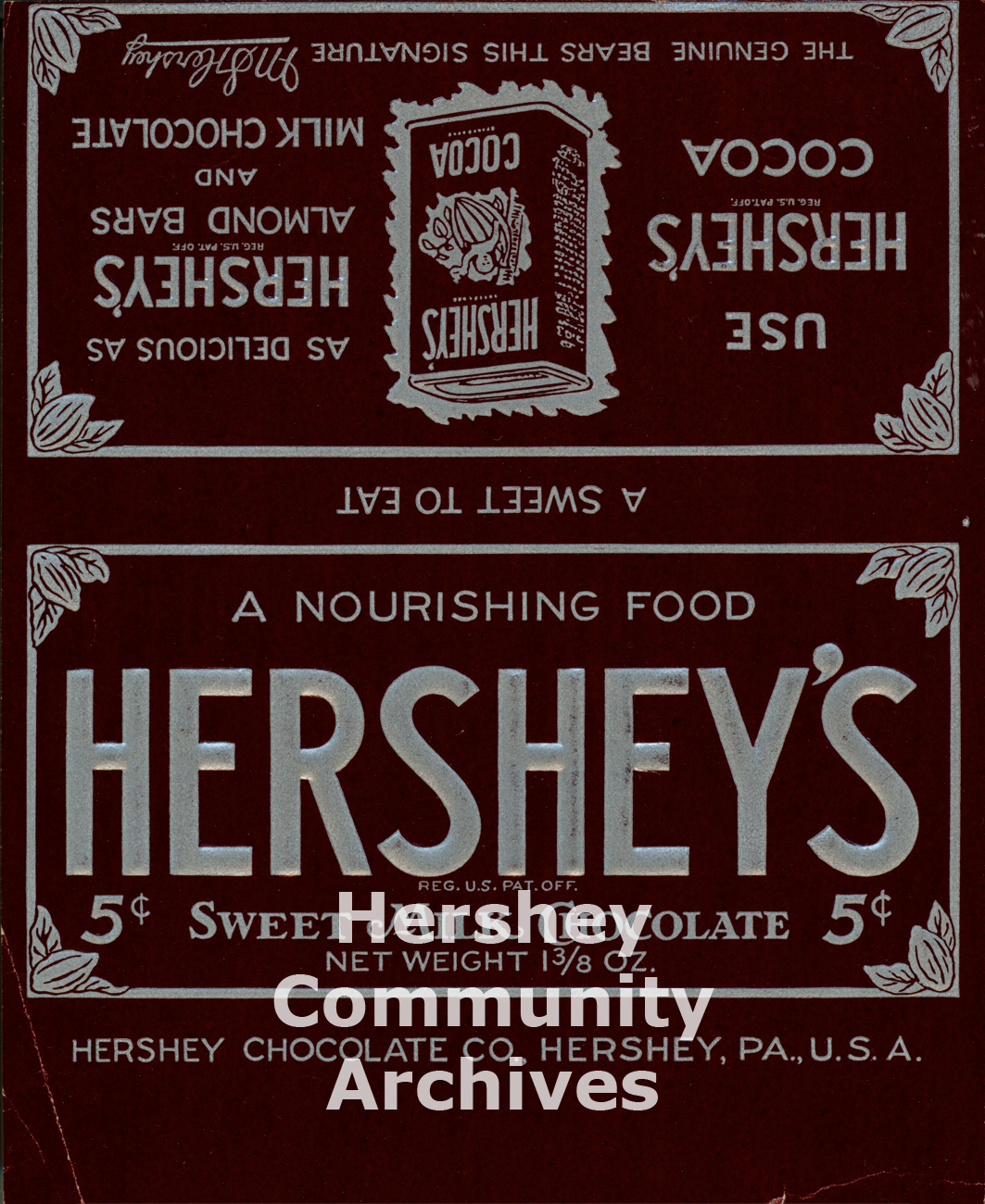This image showcases a vintage Hershey's chocolate bar wrapper, prominently featuring the label "Hershey's - A Nourishing Food" in large text and highlighting the affordable price of five cents. The wrapper, which appears to have been opened and laid flat, includes an upside-down section advertising Hershey's Cocoa, Almond Bars, and Milk Chocolate, emphasizing their deliciousness. The background of the label is a very dark brown with whitish-gray writing. At the bottom, there's a watermark from the Hershey Community Archives, indicating the historical significance of this packaging. The label also states that the product was made by the Hershey Chocolate Company in Hershey, Pennsylvania, USA. This old-school advertisement underscores the broad appeal and enjoyment of Hershey's products, positioning them as nourishing treats accessible to everyone.